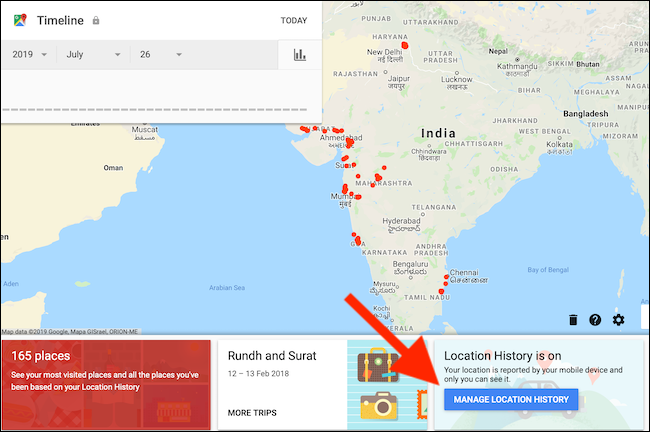This image is a detailed screenshot of the Maps application on a mobile device, capturing a user's travel history in India. Dominating the screen is a map clearly displaying India with the surrounding bodies of water - the Bay of Bengal to the east and the Arabian Sea to the west. Various red check marks are present across the map, highlighting specific locations the user has visited. 

In the top left corner, the word "Timeline" is prominently displayed, indicating that this view is part of the application's timeline feature. The date "July 26, 2019" is marked, showcasing a specific day’s travel activity, along with a summary that the user has visited 165 different places. An on-screen note reads: "See your most visited places and all the places you've been based on your location history,” suggesting that the application has meticulously tracked and documented the user’s movements.

The map reveals a trail of check marks along India's west coast, a few in the northern region around New Delhi, and several on the east coast near the Bay of Bengal. A distinctive red arrow points towards a blue button labeled "Manage Location History," possibly included for instructional purposes, directing another user on how to control or review their own location data.